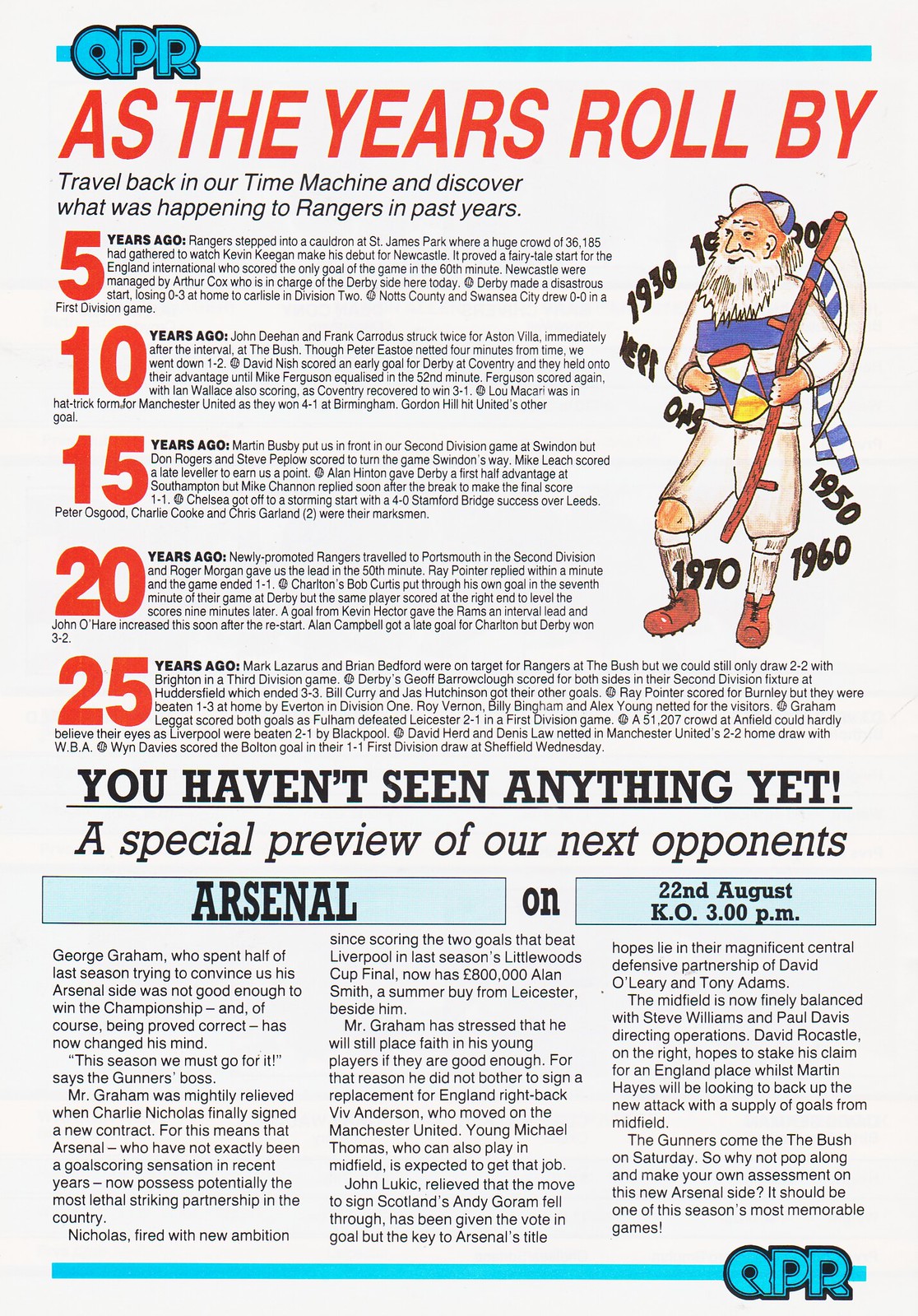This is a color image of what looks like a page from a soccer program, set against white paper. Dominating the top is a prominent blue band, with "QPR" in bold blue letters on the left. Just below, in very large red text, it reads "As the years roll by," followed by a black subtext that invites readers to "travel back in our time machine and discover what was happening to Rangers in the past years." 

At the center-left of the page, there's a series of numbers in bold red—5, 10, 15, 20, and 25—each corresponding to paragraphs of text detailing events from those years. Just over halfway down the page, bold text announces, "You haven't seen anything yet," heralding a special preview of the next opponents.

Two blue boxes are visible: one contains "Arsenal" in bold black text, while the other displays the date and time of the match, "22nd August, 3 PM KO." On the lower right-hand corner, there is another blue line with "QPR" boldly printed.

Additionally, an image appears on the top right corner of an old man dressed in white and blue, smiling, and holding a sickle and an hourglass, surrounded by the years 1930, 1940, 1950, 1960, and 1970, lending a nostalgic touch to the page.